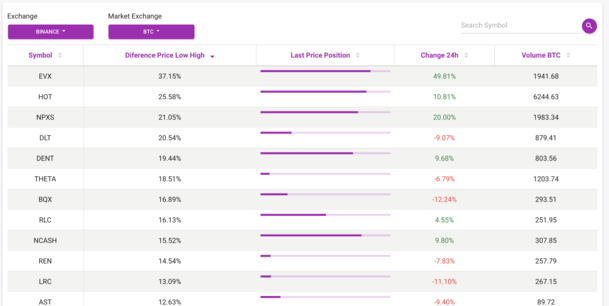In this detailed screenshot set against a white background, we see a rectangular interface dominated by black text with notable purple accents. In the upper left corner, there is a prominent purple action button labeled "Finance." To its immediate right is another action button, possibly labeled "TC," though the label is quite blurry. Directly above the "Finance" button is the word "Exchange," and to the right, the words "Market Exchange" are visible.

Below these headers, there is a detailed chart displaying various data columns. The chart is divided into sections that read from left to right: Symbol, Difference, Price, Low, High, Last Price Position, Change in 24 Hours, and Volume BTC. 

In the upper right corner of the screenshot, a purple circle encloses a magnifying glass search icon. Adjacent to this is a white search box with the placeholder text "Search Symbol."

On the left side of the chart, you can see a list of cryptocurrency symbols arranged vertically from top to bottom: EVX, HOT, NPXS, DLT, and DENT.